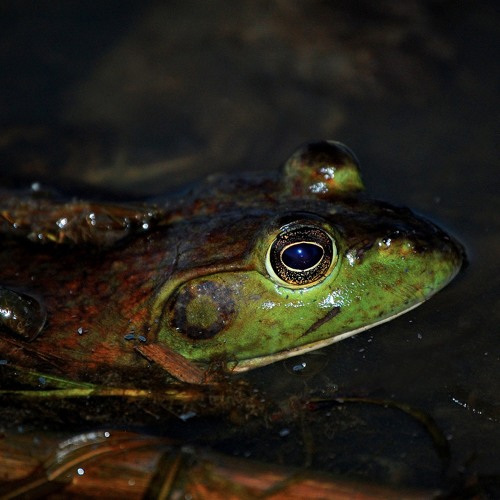A bright green frog emerges from murky, brown water, its glistening body partially submerged. The frog, prominently captured in a side profile looking to the right, stands on a twig adorned with a few leaves and hints of fuzzy moss or pond scum, localized more towards the bottom left of the image. Its vivid green face contrasts sharply with the dark, opaque water and reveals a large, golden-blue circular eye with a distinct solid blue pupil. Surrounding the eye is a horizontal oval shape adding further detail to its mesmerizing gaze. The frog's body transitions into a reddish-brown hue mixed with green patterns towards the back, suggesting a wet, shiny texture. The scene around the frog is blurred and indistinct, contributing to a mysterious ambiance with the occasional visibility of submerged rocks and plant roots in the background.